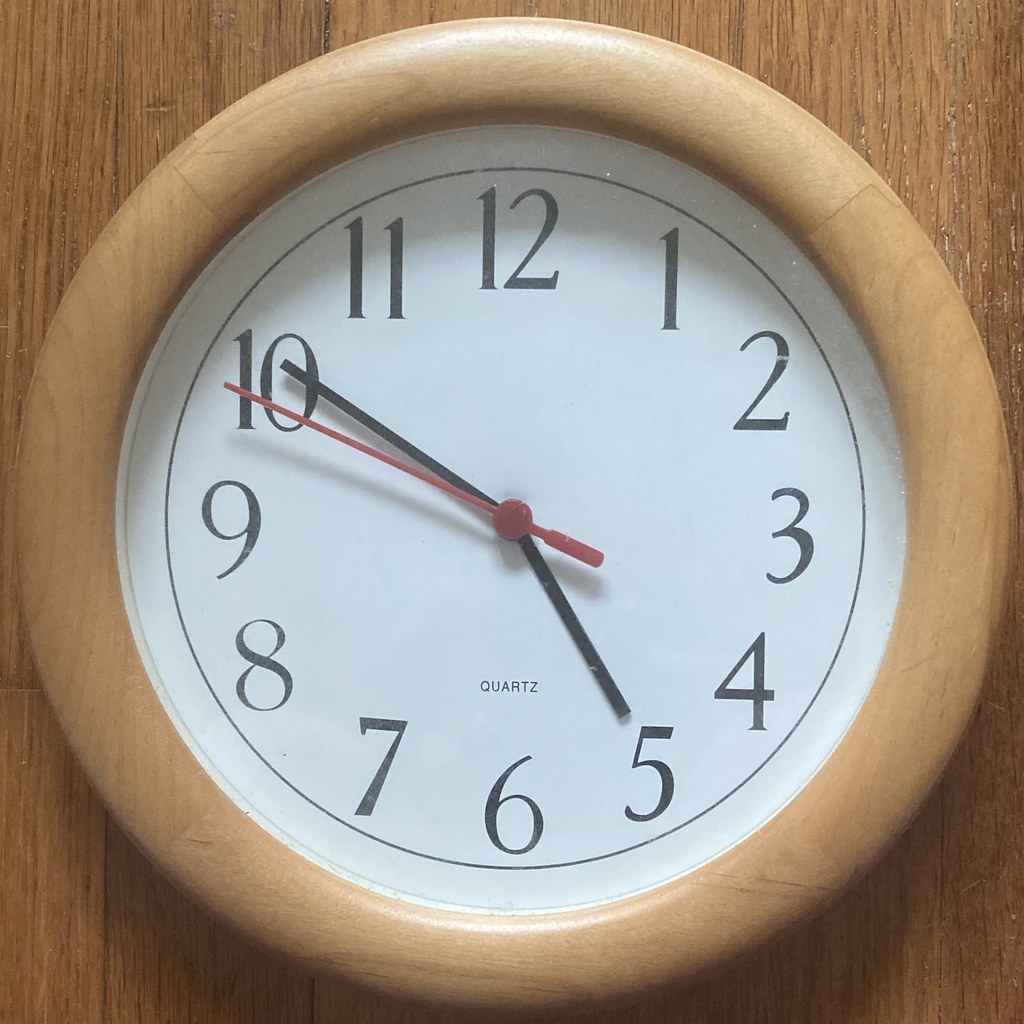The image depicts a wall clock mounted on a lighter brown wall adorned with subtle black lines running through it. The clock, encased in a glass cover, features a circular frame with a lighter brown hue tinged with a hint of green. The frame appears to be segmented into distinct sections encircling the clock face. The clock face itself is neatly inscribed with black numbers from 1 to 12, each marking their respective hours. Notably, there is a small sketch mark situated at the bottom right of the clock face. The hour hand is pointing at 5, while both the minute and second hands are directed at 10. The clock is labeled with the word "quartz," indicating its type.